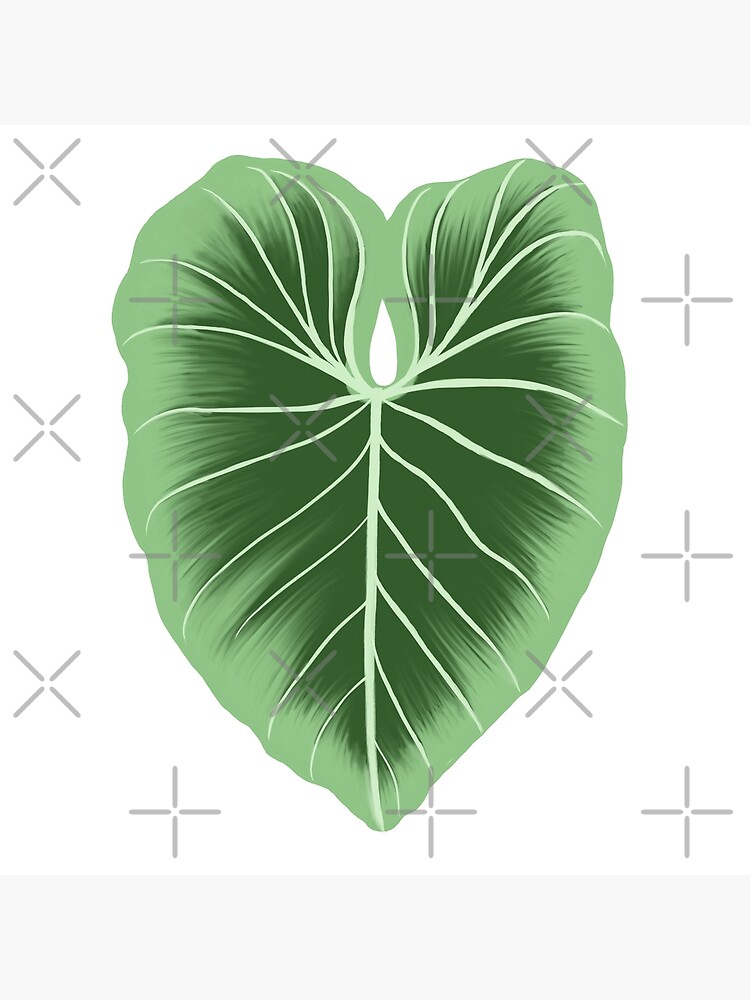This image features a detailed illustration of a heart-shaped, tropical leaf set against a white background adorned with randomly placed gray X's and plus signs. The leaf, potentially resembling an elephant ear or monstera leaf, displays a gradient of green hues. The outer edges are light green while the inner portion is a darker green. Adding to its visual depth, the veins of the leaf stand out in a light mint green, curving elegantly from the center toward the edges and tip. Near the top, the leaf has a small teardrop-shaped gap. This vector-style illustration, with its vibrant colors and watermarked background, suggests a stock image appropriate for graphic design use.